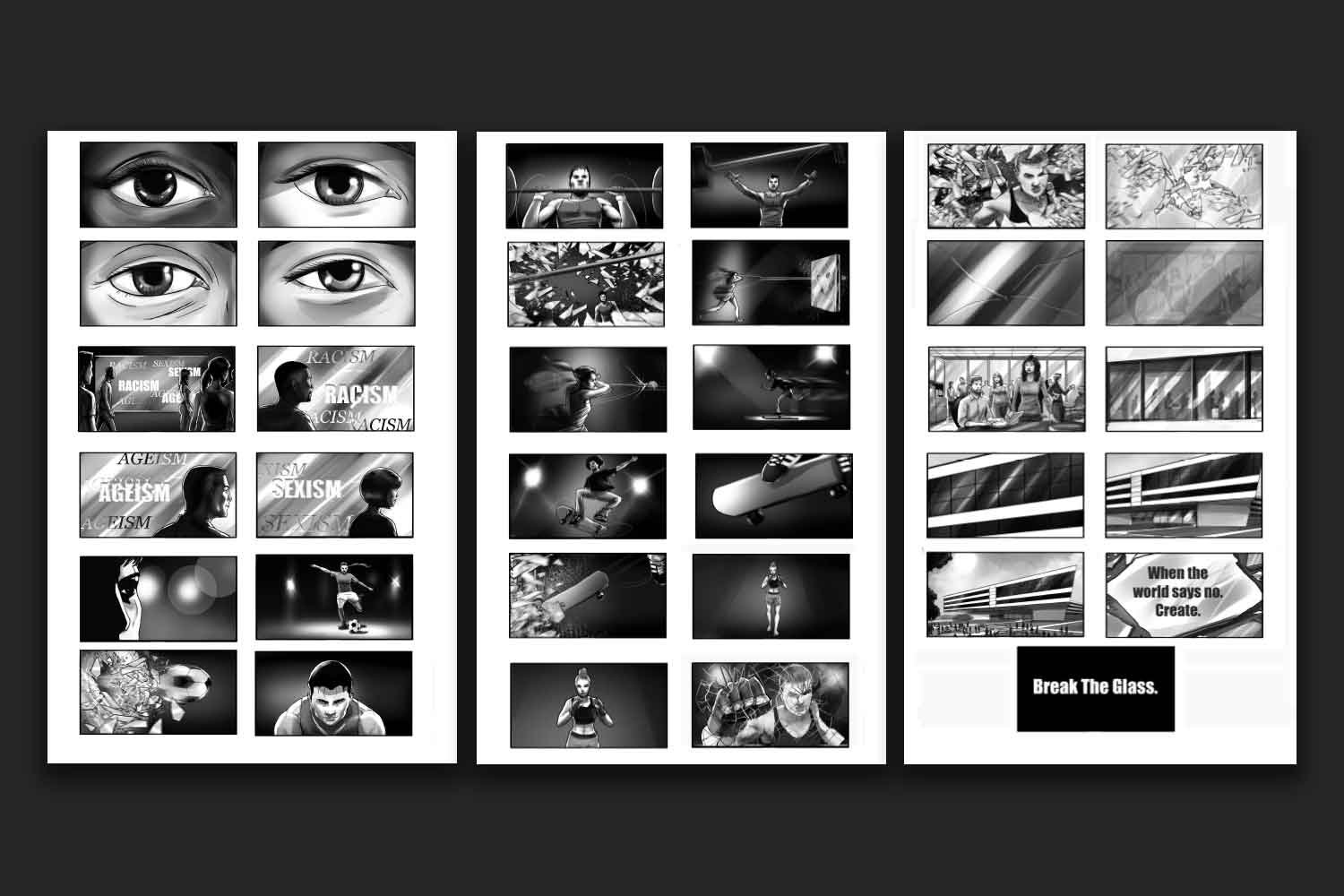The image comprises three full pages of comic-style panels, each intricately detailing various scenes. The leftmost page features a series of close-up panels focused on people's eyes, followed by middle panels that starkly present the words "racism," "ageism," and "sexism." Below these, there is a dynamic sequence of panels showcasing a person actively engaged in playing soccer.

The central page shifts its focus to physical and athletic feats, illustrating someone lifting weights and dramatically throwing their barbell, alongside other vigorous activities such as playing tennis, skateboarding, and kickboxing. 

The rightmost page introduces an assortment of intense, action-packed imagery, including depictions of breaking glass. The visual narrative culminates with a poignant message at the bottom of the page that reads, "When the world says no, create." This is followed by a directive in bold white text set against a black backdrop: "Break the glass." Unconventionally laid out, the panels might be interpreted as storyboard frames from an animation, emphasizing themes of defiance and creativity against societal oppressions.